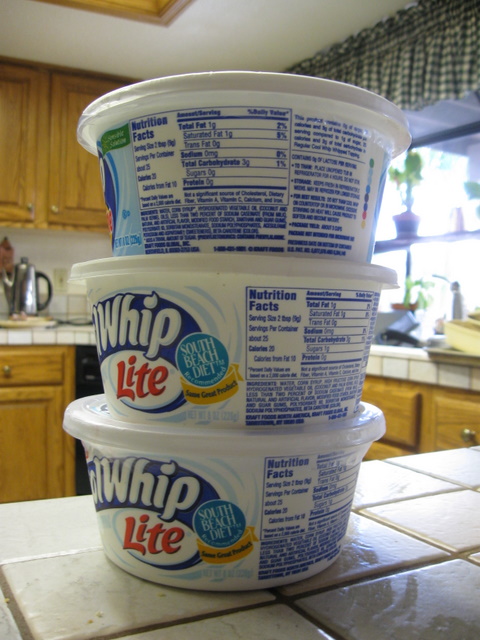A real photo captures three Cool Whip Light tubs stacked atop one another on a white tile surface in a kitchen. The bottom tub is rotated to display part of the nutrition label, which prominently features "South Beach Diet" and a partially obscured "Cool Whip Light." The middle tub is slightly more rotated to the left, revealing more of the nutrition label but still showing a portion of the front banner. The top tub is fully rotated, exposing the entire nutrition label, the list of ingredients, and additional product information, likely indicating the presence of bioengineered ingredients. The background showcases brown kitchen cabinets.